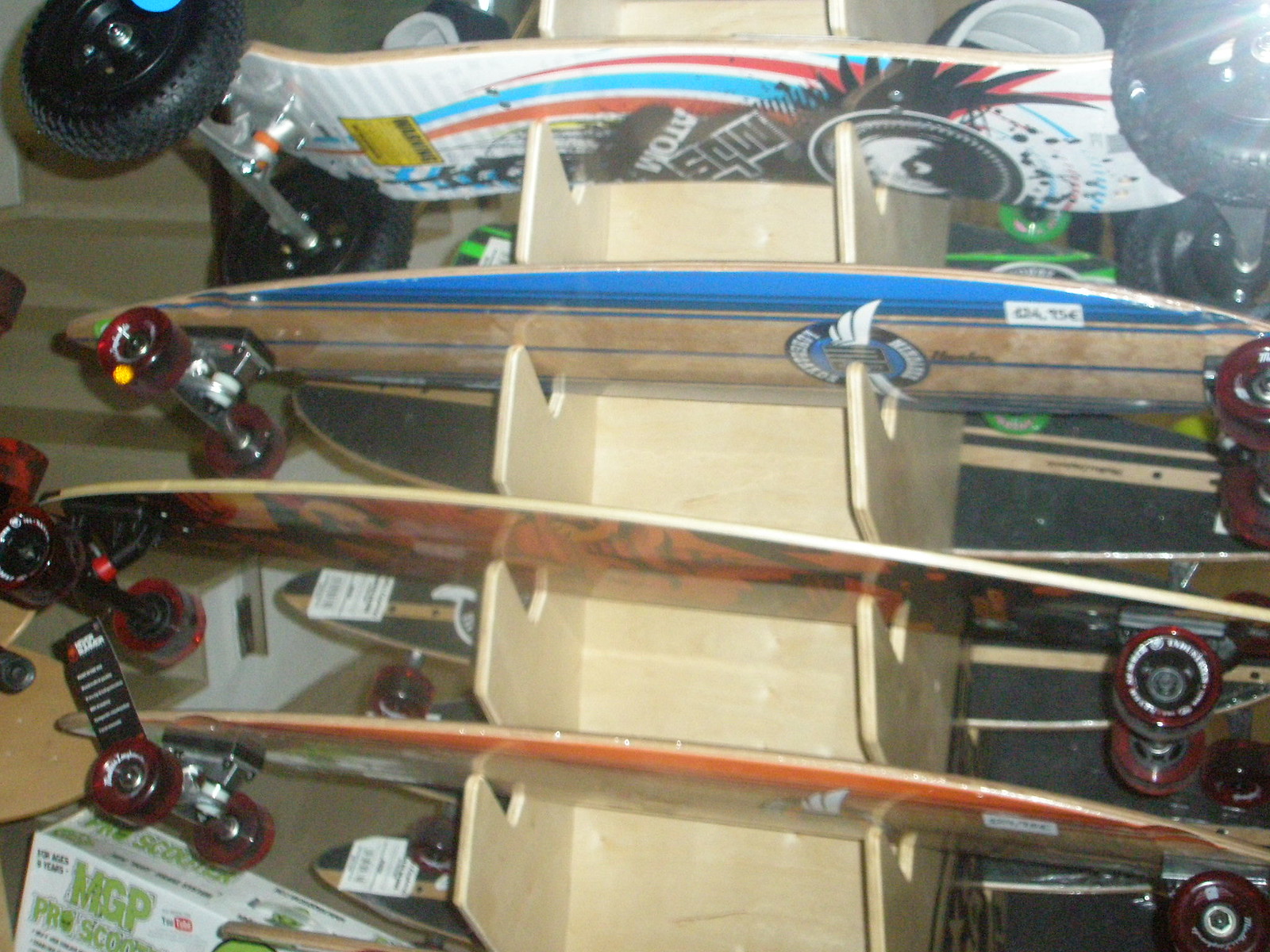The image captures the inside of a skateboard shop, featuring a light brown, tan rack holding a display of four longboards, which are larger than standard skateboards. At the top of the rack is a vibrant, multicolored longboard with a white base and accents of red, yellow, and blue, equipped with large black wheels and chrome and orange trucks. Below it, there are three more longboards with varying designs and colors, predominantly wood, blue, and orange, all featuring either chrome or black trucks and burgundy or red wheels. The background shows several other skateboards with visible grip tape, though their details are obscured. Additionally, a white box with green writing, whose text is indiscernible, is situated in the lower left corner of the image.